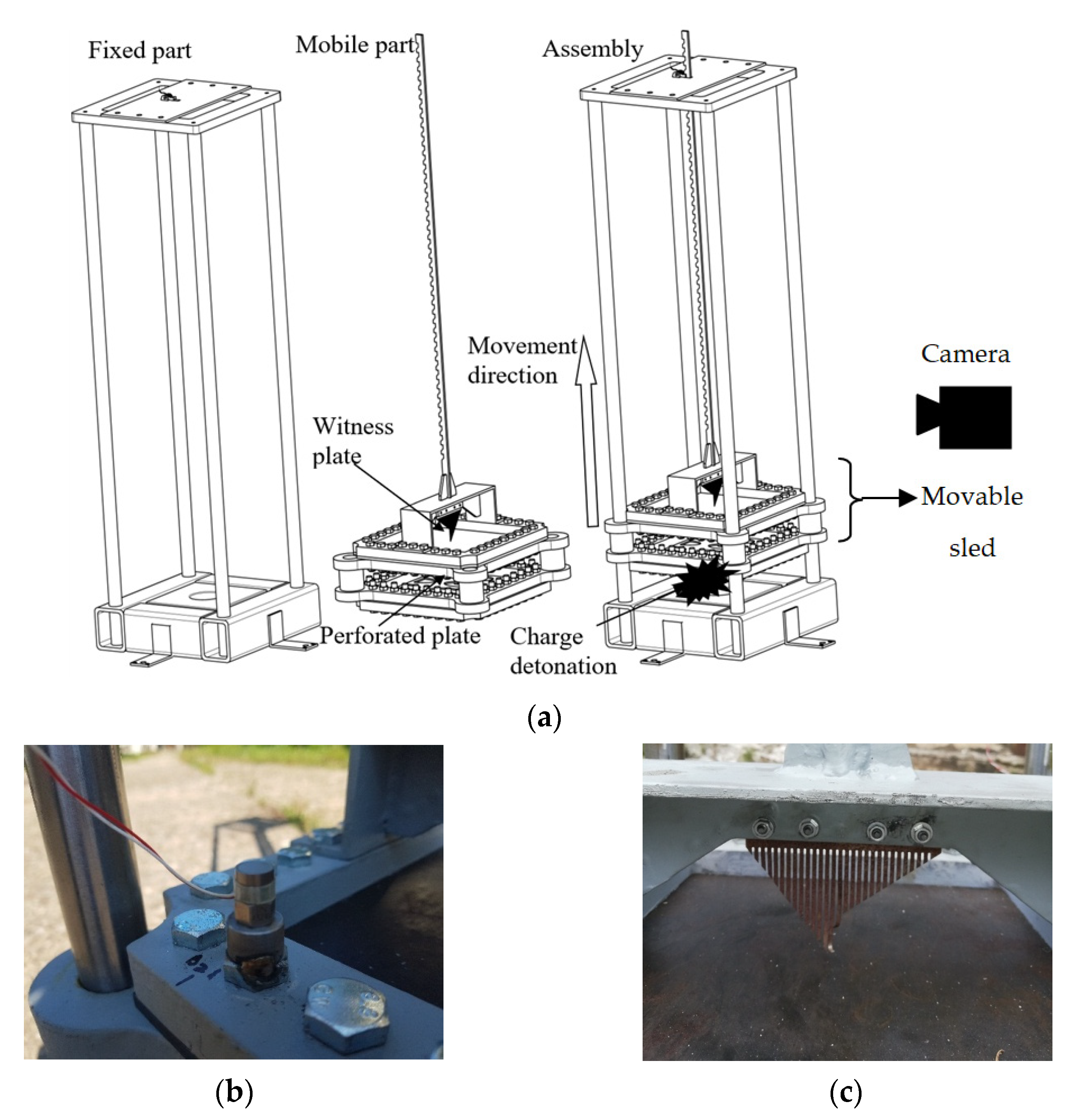The image depicts a detailed mechanical diagram, possibly for an invention, including both an illustrative drawing and photographic representations of metal components. The drawing is labeled with multiple terms such as "fixed part," "mobile part," "witness plate," "perforated plate," "charge detonation," "movement direction," "assembly," "camera," and "movable sled." The diagram is divided into two main sections: the fixed part, consisting of four vertical walls connected by top and bottom surfaces, and the mobile part, which is inserted into the fixed part and features a saw-like structure extending its length. Below the main drawing, there are two additional images labeled B and C, showing close-ups of bolts and the relative position to the ground, highlighting assembly details. The fixed part, designed to protect the internal components, is shown connecting to the ground, emphasizing its stability. The assembly view illustrates how the mobile part fits within the fixed part, aligning with terms like "charge detonation" and indicating an upwards movement direction. The color scheme includes browns and grays, aiding in the differentiation of components. The intricate diagram serves as a comprehensive guide to assembling this potentially complex and functional part.